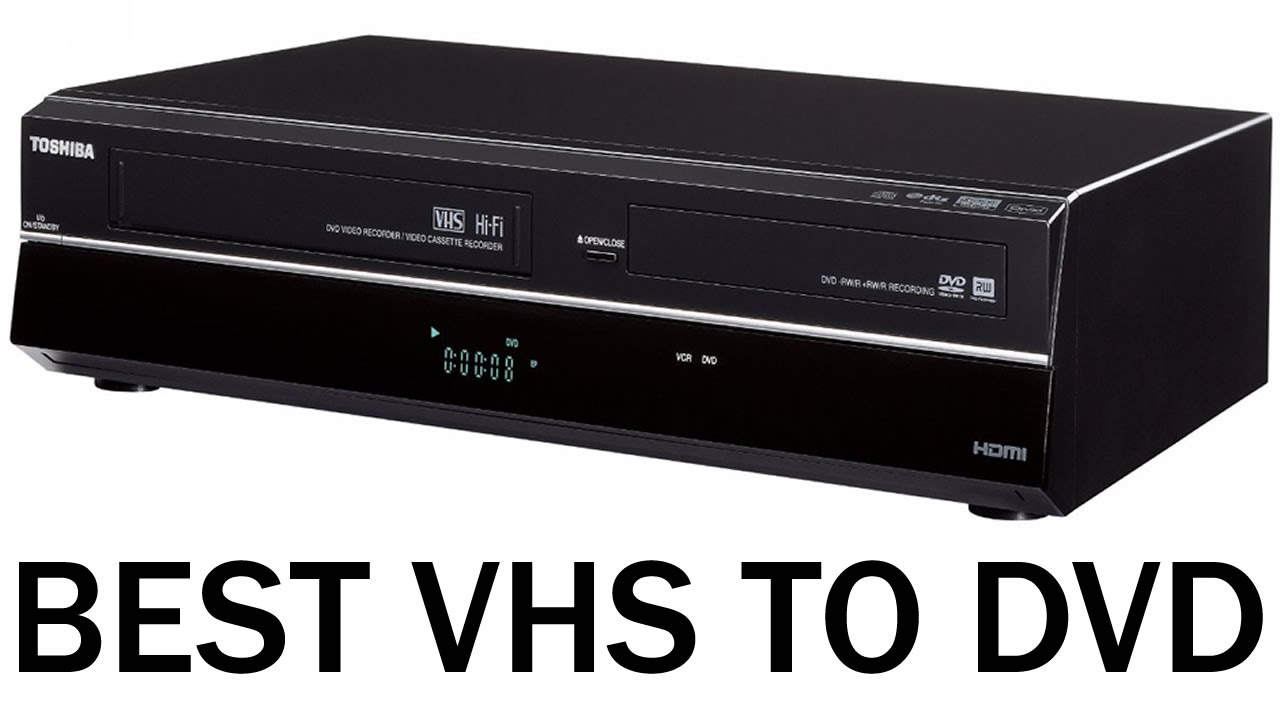This image features a black Toshiba VHS and DVD combo player set against a white background. The front of the device is demarcated clearly: the VHS slot is on the left side and the DVD slot on the right. Each slot is labeled accordingly with "VHS" and "DVD" in white text. Below these slots is a digital display panel that likely indicates playback information for DVDs, as similar functionality is not typical for VHS tapes. This piece of equipment appears to be from the late 1990s or early 2000s when such combo players were popular for transitioning media from VHS to DVD formats. Additional white text on the device includes "VHS Hi-Fi" on the upper left and "HDMI" on the bottom right corner. Underneath the display panel, in black text, is the phrase "Best VHS to DVD," suggesting it could have been used for advertising purposes. The digital display on the panel shows "00:00:08" alongside icons for VCR and DVD functions, adding to the comprehensive labeling of its features.